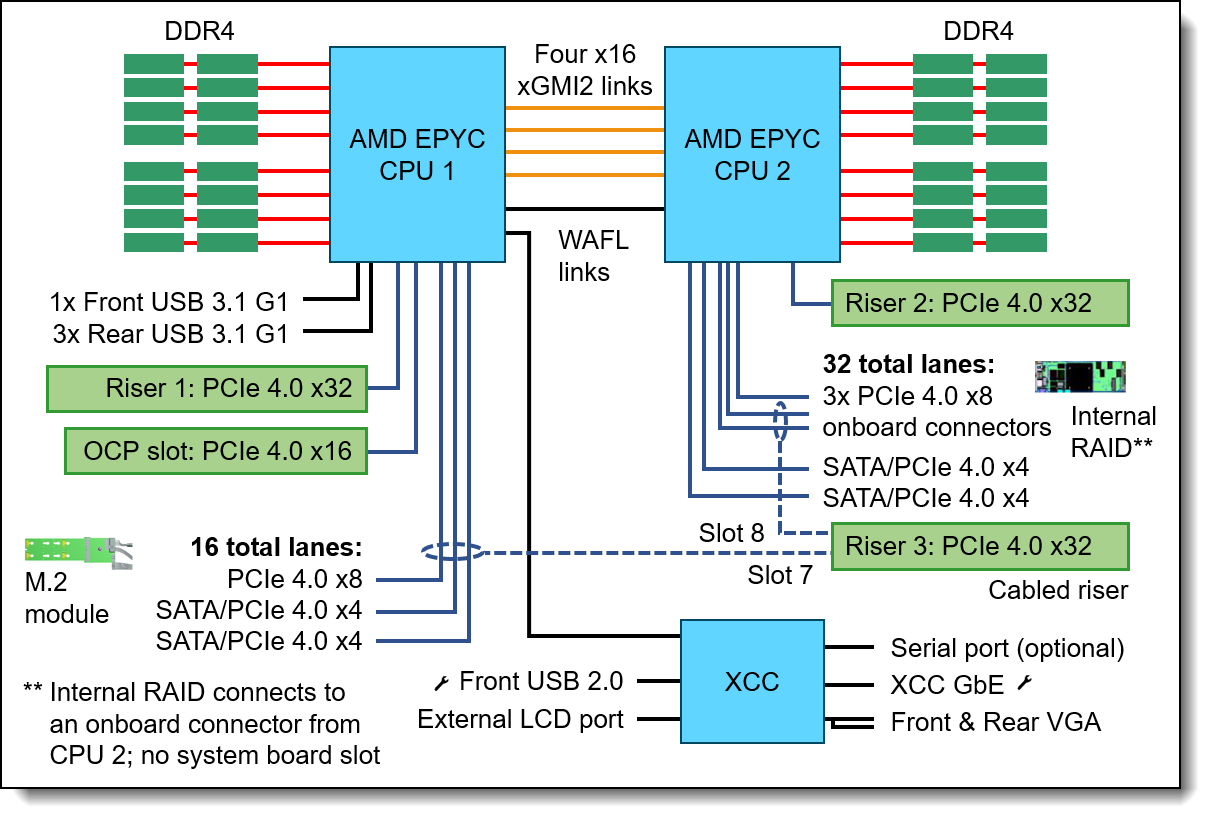The diagram illustrates the intricate layout of a high-performance server or supercomputer motherboard, depicting detailed connections between multiple components. Central to the diagram are two AMD EPYC CPUs, labeled as CPU 1 and CPU 2, each connected to 16 DDR4 RAM modules via red cables. The DDR4 modules are represented by green boxes with black lettering. Additional intricate components include various slots and connectors such as PCIe 4, SATA, RAID, M.2 modules, and risers. A notable feature is the internal RAID setup that links directly to an onboard connector from CPU 2, bypassing the system board slot. Lines and connectors meticulously detail the links between these components, emphasizing the complexity and capacity of the system. This comprehensive diagram underscores the advanced architecture typical of server-grade or supercomputer hardware.